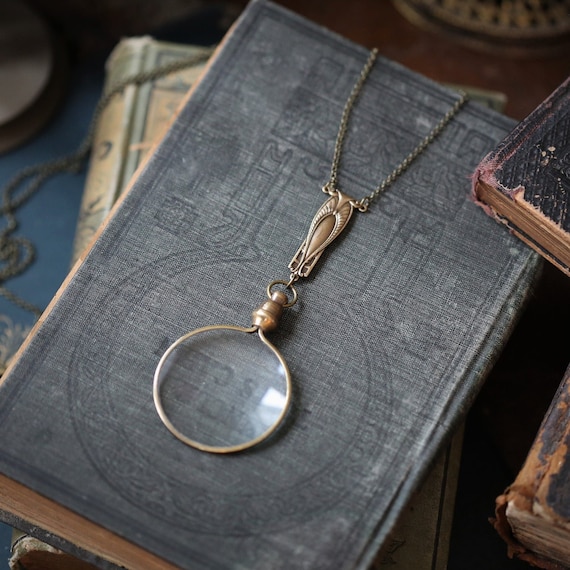In this evocative photograph, a collection of antique books is carefully stacked, showcasing their age and character. At the forefront, a weathered hardcover book with a rich blue cover lies on top, its pages tinged with a tannish brown hue from years of existence. Draped over this book is an intricate necklace, featuring a greenish chain and a striking gold centerpiece that resembles a zipper. This unique pendant connects to the base with a gold loop, eventually forming a circular design that frames a piece of glass, reminiscent of a magnifying glass. To the right, the worn edges of two leather-bound books peek into the frame, their covers showing signs of deterioration, adding to the nostalgic charm of the scene. The photo captures a moment where vintage literature and delicate jewelry converge, evoking a sense of history and timeless beauty.